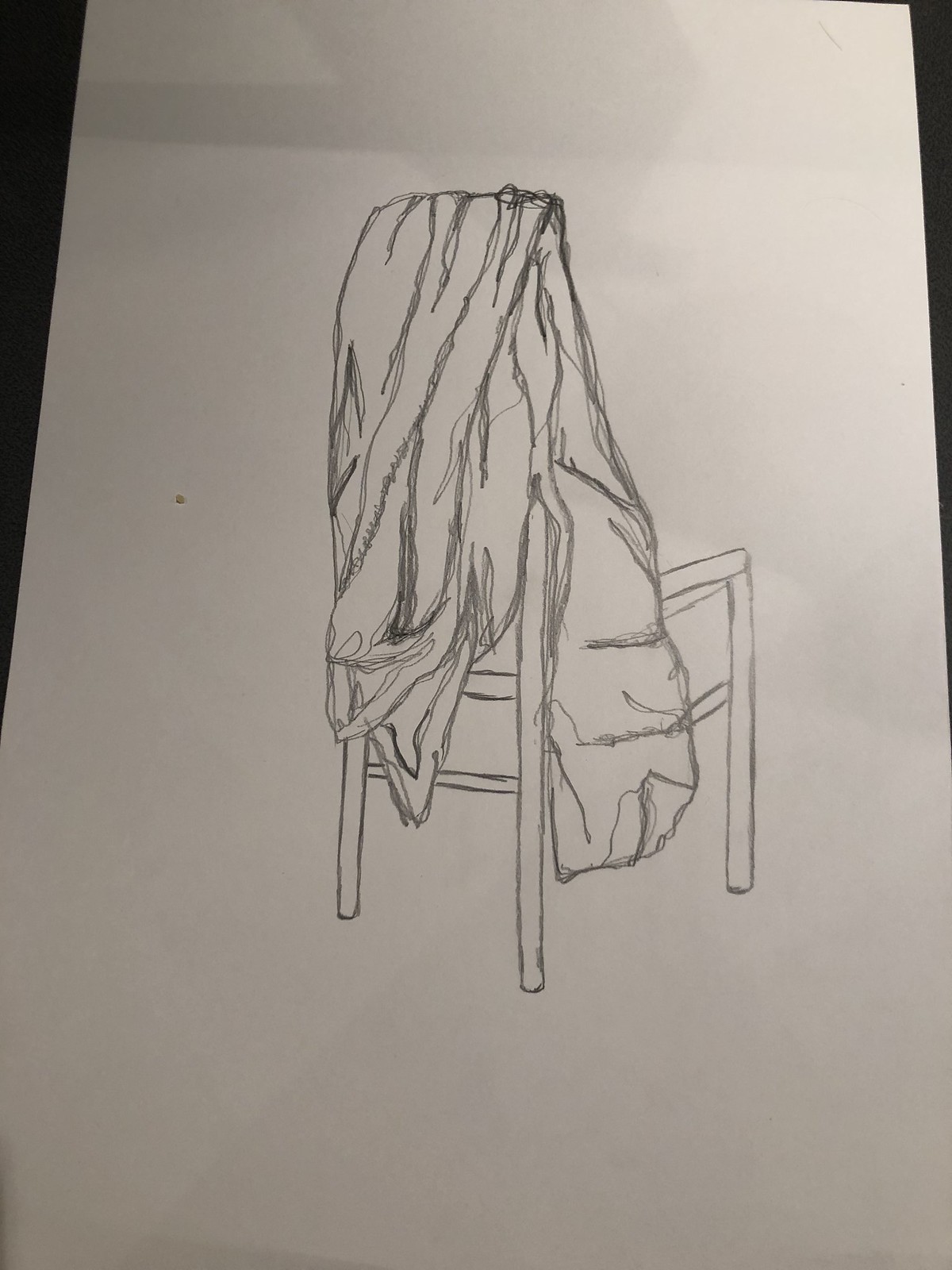The image depicts a detailed pencil sketch on a long white piece of paper, which is approximately the width of standard notebook paper but about two to two and a half times its length. The paper is placed on an indistinct black surface, possibly a table, though the background is not discernible. Centered on the paper is the hand-drawn image of a wooden kitchen chair, characterized by its high back and structural simplicity, with visible supporting bars and three legs clearly shown. Draped over the back of the chair is a large, fluffy coat or parka with big sleeves, drawn with evident folds yet minimal shading. The garment hangs at an irregular angle, suggesting a realistic practice in capturing the dynamics of fabric over furniture. The drawing is approximately 7.5 inches (15 centimeters) in height and is rendered with a soft pencil, giving it a delicate, understated appearance.